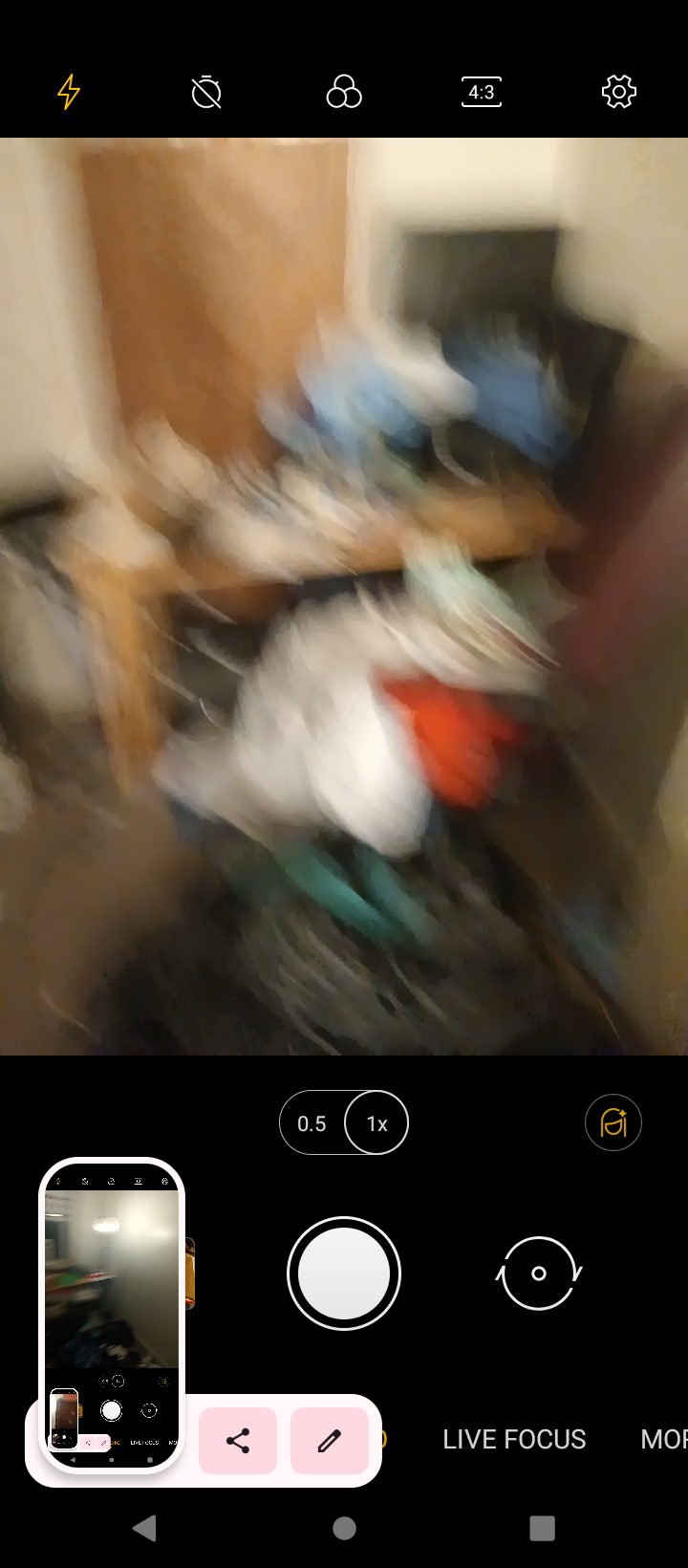The image displays a phone screen showcasing a blurry, low-resolution picture, giving the impression of motion. At the center of the screen, indistinct shapes in white and red are visible. The background reveals a light brown desk, although the details remain unclear due to the poor image quality. Below the picture, a numerical indicator reads "0.5" on the left and "1x" to its right. Further right on the screen, there is an illustration of a girl in yellow. Additionally, a yellow lightning bolt icon is present in the top-left corner of the screen.